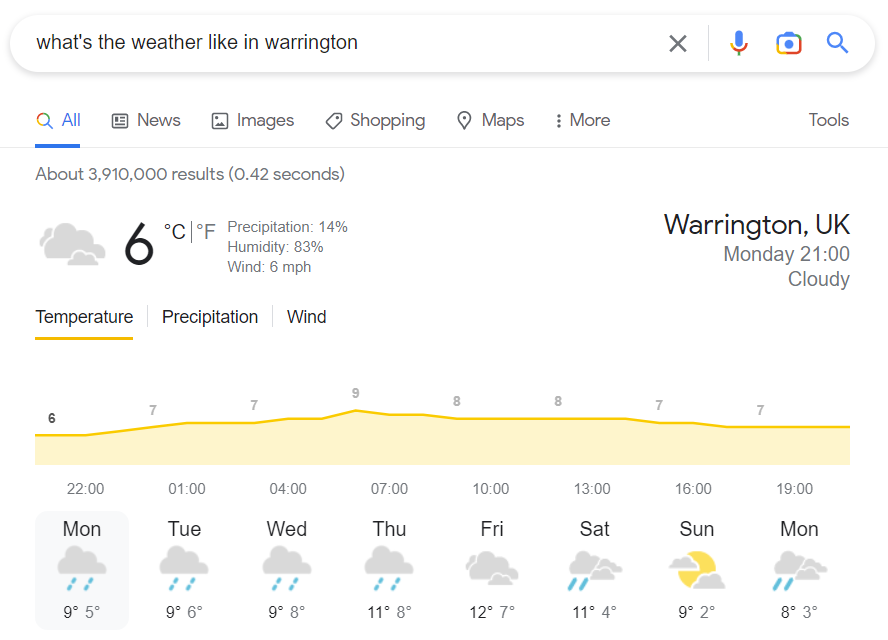The image depicts a Google search results page with a query for the current weather in Warrington, UK. The search bar displays the question, "What's the weather like in Warrington?" The resulting weather information reveals it is currently 6 degrees Celsius with 14% precipitation, 83% humidity, and wind speeds of 6 miles per hour. The time is noted as 21:00 (9 PM) on a Monday, and the weather is cloudy. A weekly weather forecast graph is also visible, with a yellow line showing temperature trends from Monday to the following Monday. The temperatures for the week are summarized as follows: 

- **Tuesday:** 9°C to 6°C 
- **Wednesday:** 9°C to 8°C 
- **Thursday:** 11°C to 8°C 
- **Friday:** 12°C to 7°C 
- **Saturday:** 11°C to 4°C 
- **Sunday:** 9°C to 2°C 
- **Monday:** 8°C to 3°C 

All temperatures are given in degrees Celsius.